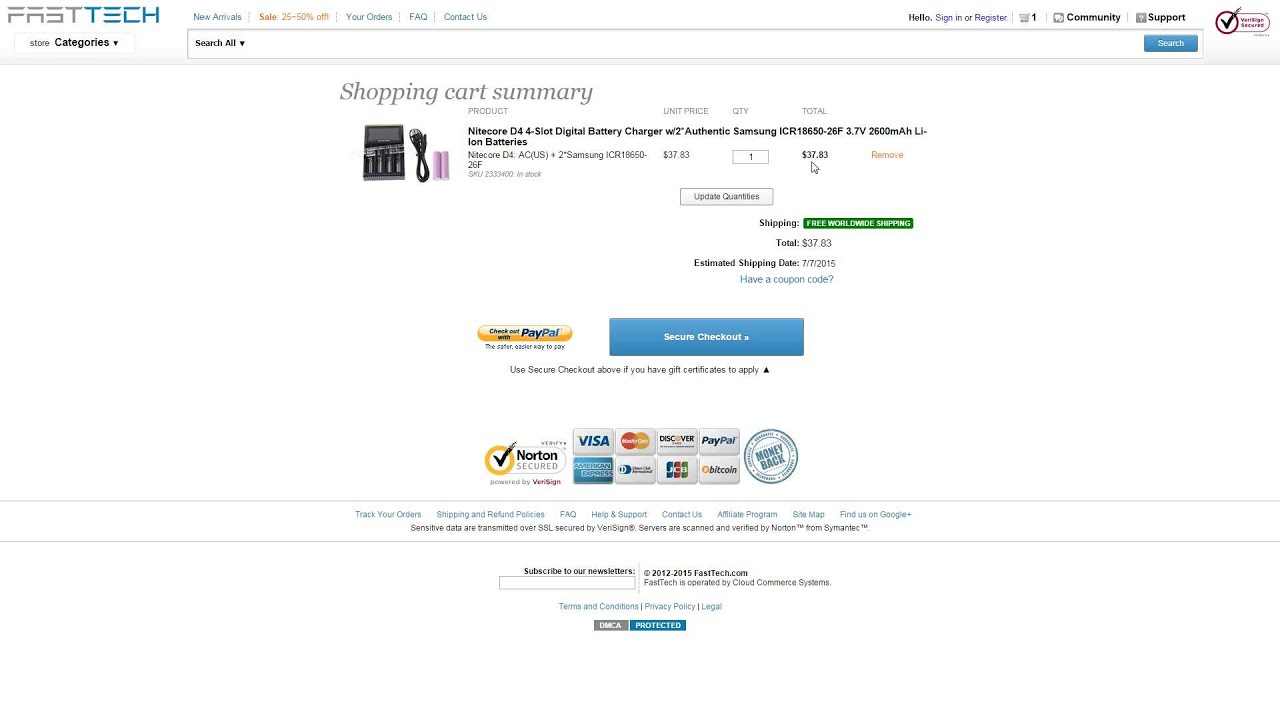Here's the refined and detailed caption for the screenshot of the website:

---

This screenshot showcases the homepage of the "Fast Tech" website. At the top, the company name is prominently displayed with "Fast" in bold, grey print, and "Tech" in a vibrant teal color. To the right, a navigation bar offers links such as "New Arrivals," "Sale 25-50% Off Your Orders," "FAQ," and "Contact Us."

In the upper-right corner, user-related options are visible, including "Hello, Sign In" and "Register" in blue-purple text. Next to these options is a shopping cart icon with a notification indicating one item. Additionally, there is a link to "Community and Support" beside a burgundy circle with a checkmark, signifying secured site credentials.

Beneath the main header, there is a store navigation menu with a "Categories" dropdown and a search bar. The search bar includes a “Search All” option with a down arrow, followed by a prominent blue banner with white text.

Below this, the "Shopping Cart Summary" is detailed against a white background, presenting the following information:
- Product: "Nitecore D4 Digital Battery Charger with 2-inch Samsung"
- Specifications: "3.7V 2600mAh Li-Ion Batteries"
- Unit Price: $37.83
- Quantity: 1
- Total: $37.83

Options to "Remove" the item and "Update Quantities" are available. Shipping is highlighted with a banner stating "Free Worldwide Shipping." The summary also includes an estimated shipping date of July 7, 2015.

At the bottom of the summary, there is a prompt to apply a coupon code and two checkout options: "Check Out with PayPal" and a blue banner for "Secure Checkout," encouraging users to proceed securely. There is also a note about using gift certificates if available.

---